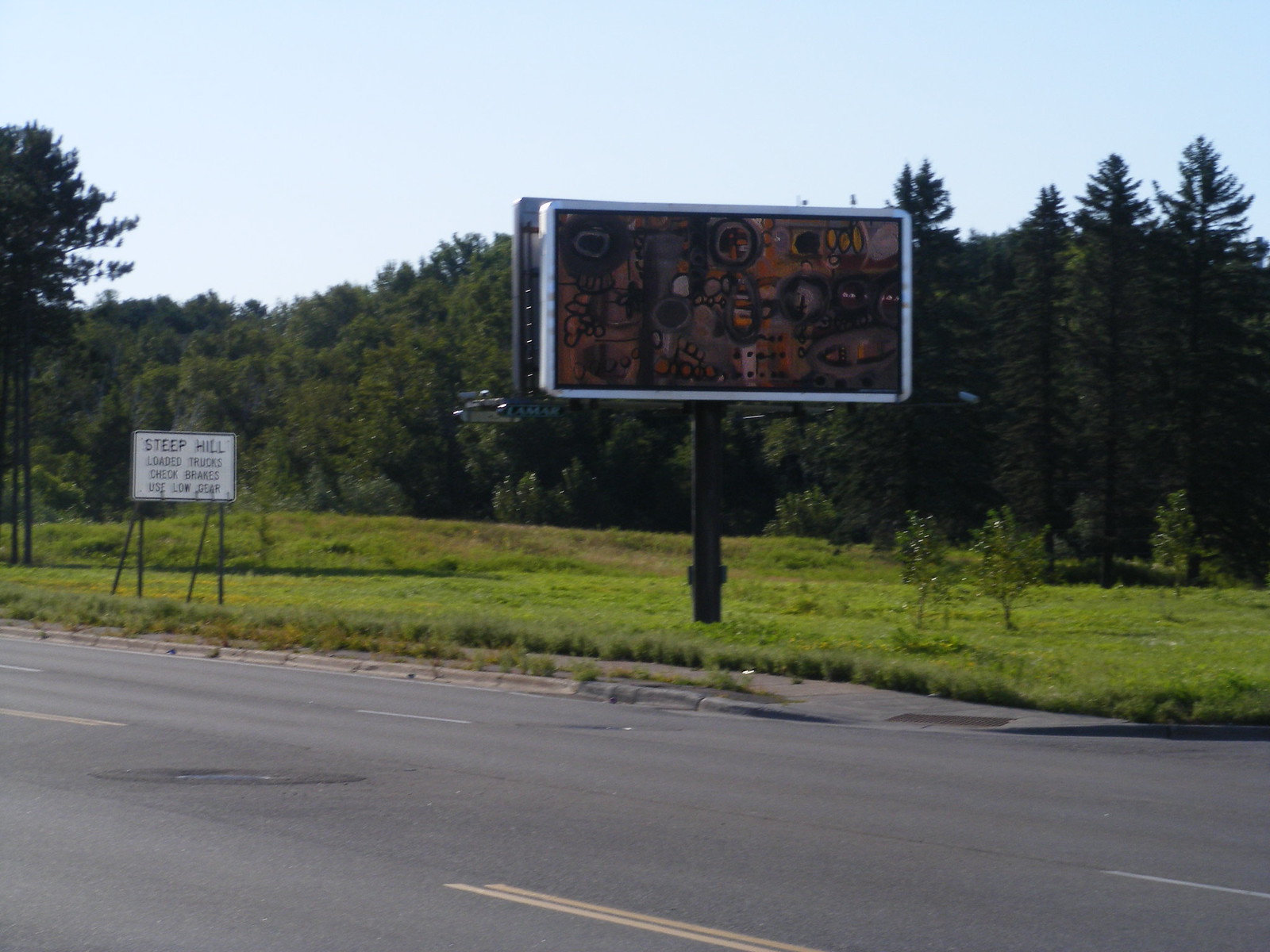A color photograph captures a scene of a blacktop road intersected by yellow lane dividers. In the background, a grassy area gives way to a tall, dense forest with myriad towering trees, all under a gray, overcast sky. Dominating the right side of the image, a black billboard has been taken over by vivid, multicolored graffiti, transforming it into an abstract canvas. To the far left, a prominent traffic sign reads, "Steep Hill. Loaded trucks, check brakes, use low gear." The absence of people, animals, buildings, and vehicles accentuates the desolation of this striking roadside vista.